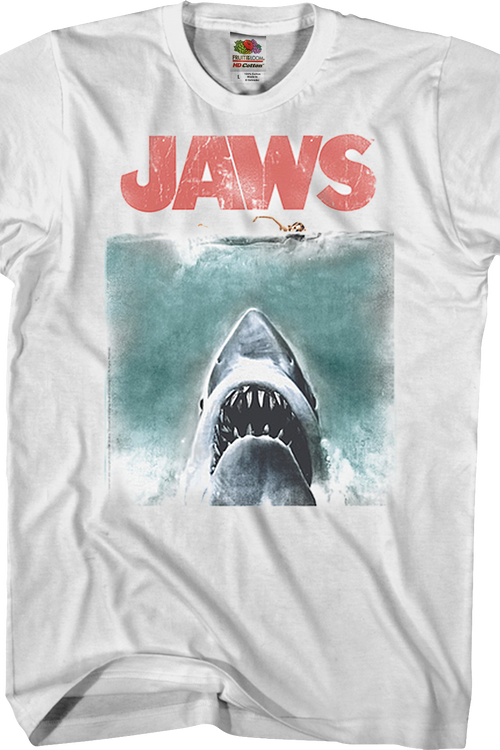This image features a detailed photograph of a white, short-sleeved Fruit of the Loom t-shirt that prominently advertises the classic movie "Jaws." The t-shirt displays the word "JAWS" in large, capital red letters at the top, crafted in a weathered, aged font that gives it a vintage feel with patches of white suggesting wear. Directly beneath the text is a striking graphic reminiscent of the movie poster: it depicts a woman swimming at the surface of the ocean with the infamous Jaws shark emerging from the depths below her. The shark is depicted with its mouth wide open, showcasing rows of sharp teeth, menacing black eyes, and visible nostrils. The overall image, including the shark and the swimmer, has a charcoaled, aged texture enhancing the retro aesthetic of the t-shirt. Though the t-shirt looks fairly new and unworn, it appears slightly folded. The garment size is identified as large, confirmed by the visible Fruit of the Loom label featuring their classic logo with various fruits.